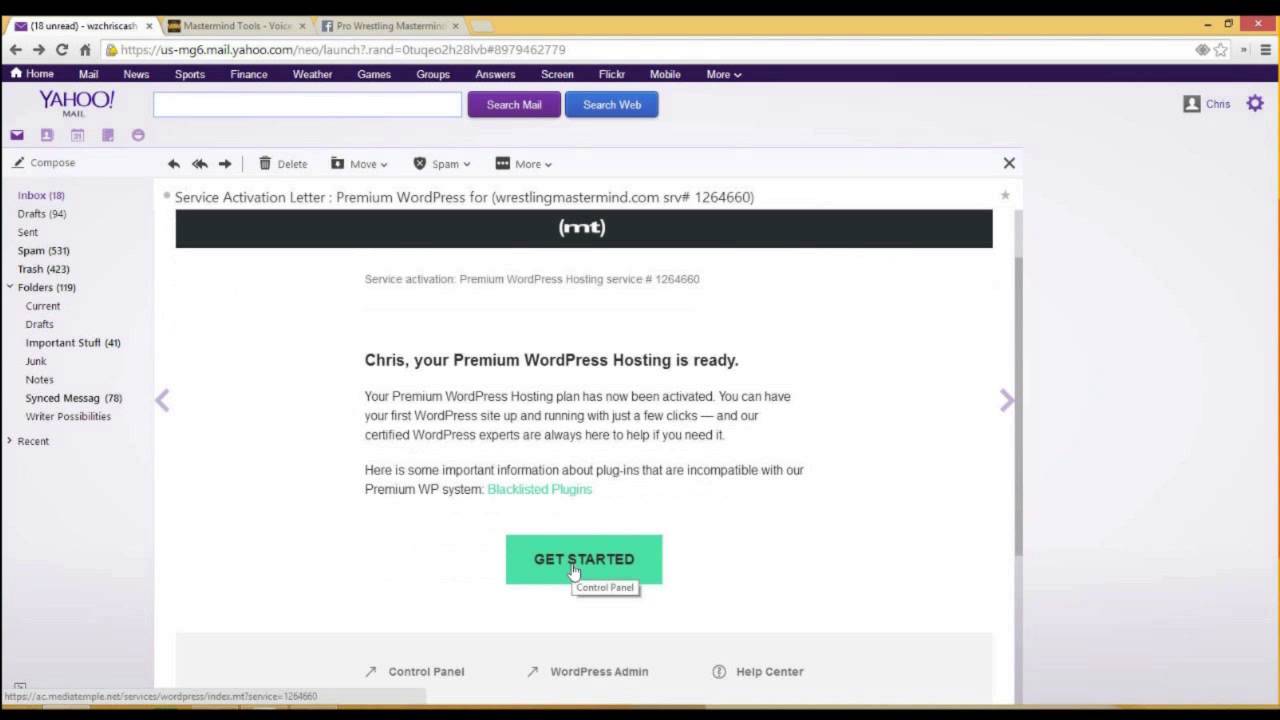The image shows a computer screen with a screen capture of a browser displaying three open tabs. The active tab is purple, featuring the YouTube logo with a notification indicating "18 unread" messages, followed by additional text. The other two tabs are labeled "Mastermind Tools" and "Facebook Pro Wrestling Mastermind."

The visible page on the screen appears to be the Yahoo Mail homepage, featuring a black banner with navigation options including Home, Mail, News, Sports, Finance, Weather, Games, Groups, Answers, and More. The user is currently in the Mail section, which is evident from the visible "Search Mail" field with a purple search button and a "Search Web" option.

The inbox is displayed with one open email titled "Service Activation Letter from Premium WordPress – Wrestling Mastermind," which contains a message indicating that the user's premium WordPress hosting is ready. There is a prominent call-to-action button labeled "Get Started," with the cursor hovering over it, suggesting the user is about to click to proceed with the setup.